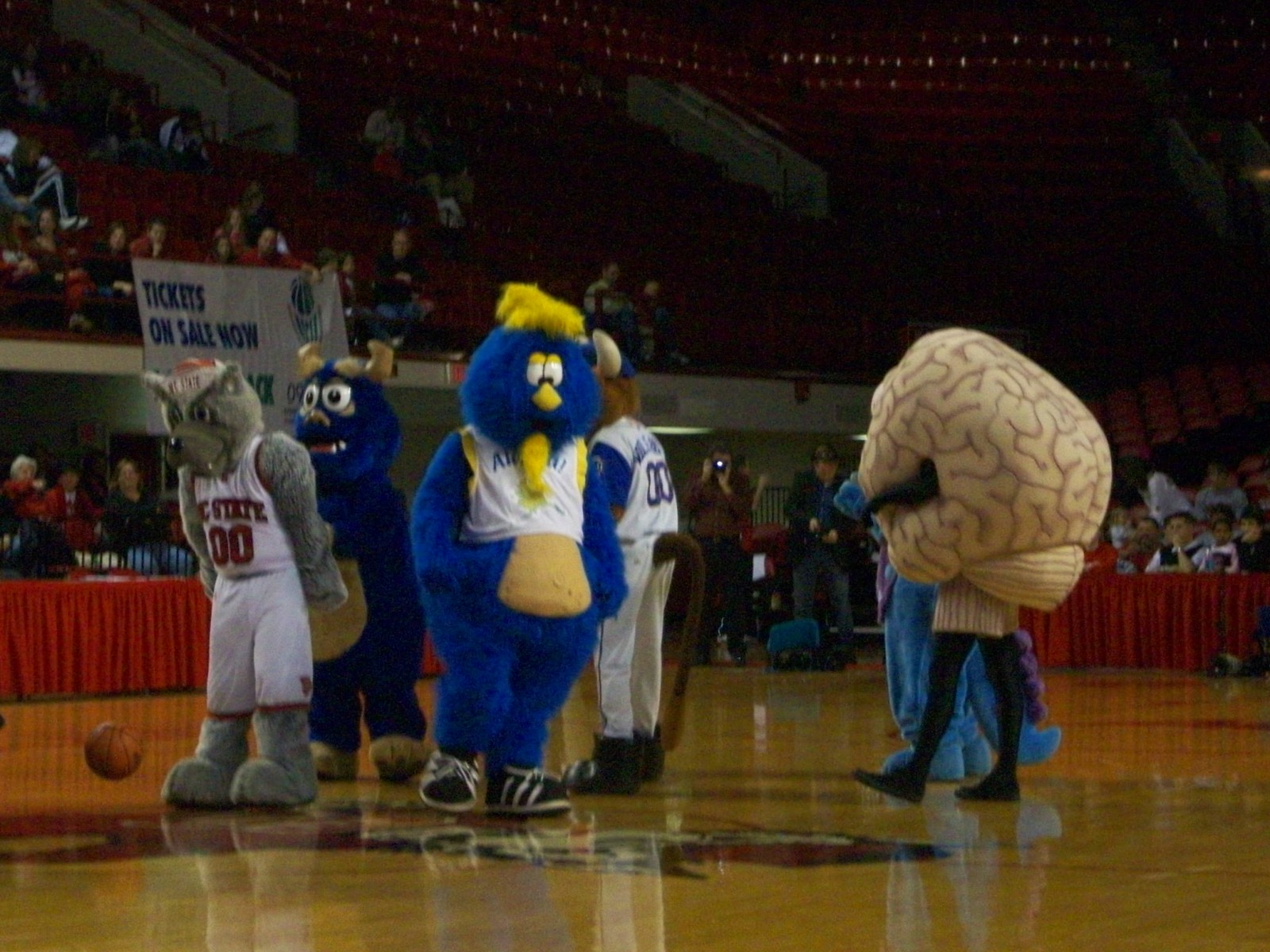The image captures a vibrant scene on a basketball court featuring six mascots at a game in a large stadium, filled with fans in the bleachers and officials seated at tables draped in red cloth. In the center of the photo, the mascots are grouped with four on the left and two on the right, one of whom is partially hidden. From left to right, the first mascot is a gray wolf in a white jersey with red lettering and white shorts. Second is a dark blue monster with small tan horns and a tan belly. Next, positioned closer to the viewer, is a slightly brighter dark blue, yellow-haired monster with a yellow nose, yellow beard, and a white, blue, and yellow jersey that ends around its waist, revealing a large yellow belly and enormous black shoes. Behind this monster stands a bull mascot, characterized by dark brown fur, a long tail, and light colored horns, dressed in a baseball uniform. To the right, there is a large cream-colored brain mascot with black arms and legs. Finally, completing the lineup, a blue dinosaur or monster with purple detailing and a long blue tail can be seen peeking out.